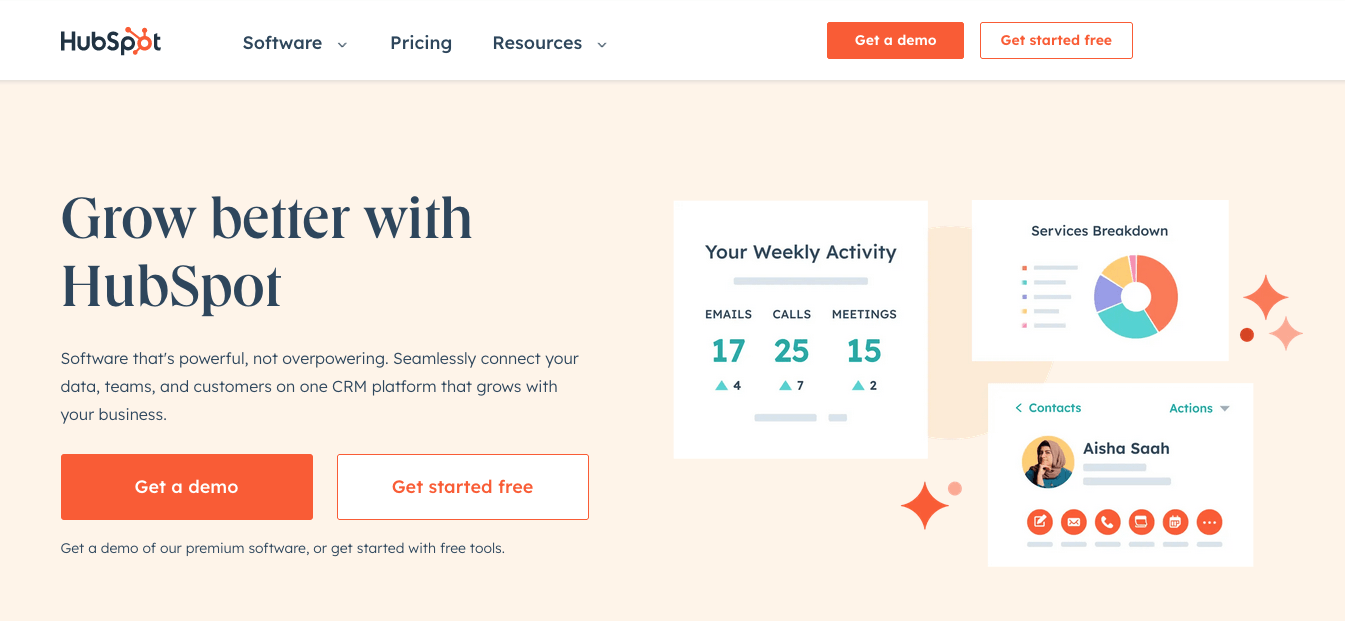This image is a screenshot from the homepage of the HubSpot website. At the center of the page, there is a large, prominent banner featuring the tagline "Grow Better with HubSpot." The text underlines the theme, "Software that's powerful, not overpowering. Seamlessly connect your data, teams, and customers on one CRM platform that grows with your business."

Directly below this central message, there are two notable call-to-action buttons. The first button, with white text on an orange background, prompts visitors to "Get a demo." The second button, featuring orange text on a white background, encourages users to "Get started free." Below these buttons, a supportive message explains the options: "Get a demo of our premium software or get started with free tools."

To the right of the central text, there are three representative images, each showcasing different features of the HubSpot platform. The first image displays a weekly activity dashboard with metrics for emails, calls, and meetings. The second image is a pie chart labeled "Services Breakdown," though the specific services are not visible. The third image is a sample contact sheet for a person named Ayesha Saw.

At the top of the homepage, the HubSpot logo is prominently displayed, with "H-U-B-S-P-O-T" written out and "Spot" highlighted in orange with multiple arrows radiating from it. Adjacent to the logo are navigation buttons for "Software," "Pricing," "Resources," and the same "Get a Demo" and "Get Started Free" buttons seen in the central banner.